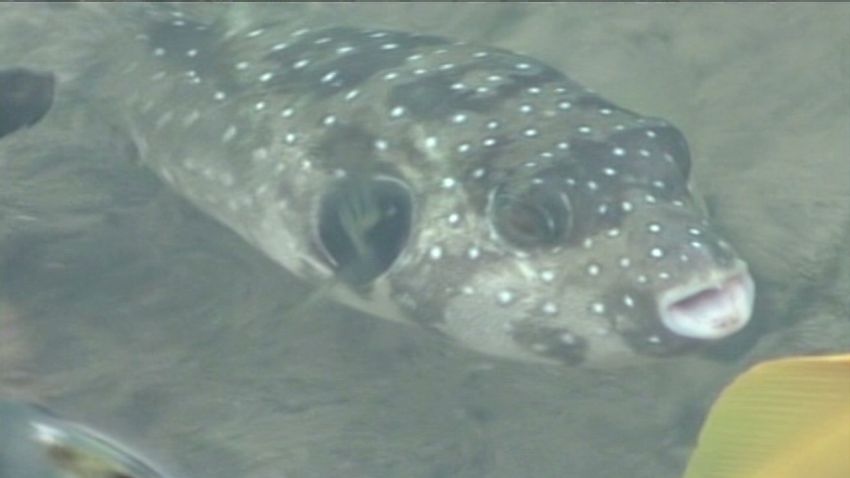The image captures a large fish underwater, most likely in natural light, although artificial light cannot be ruled out. The photograph, horizontally rectangular and without a border, has a background of indistinct sand. The fish is positioned diagonally, with its tail in the upper left-hand corner and its open mouth pointing towards the lower right-hand corner. It has a thick body that is primarily gray with patches of brown and is adorned with numerous white dots and specks across its body and face. The water is murky, imparting a grayish-greenish-black hue to the entire scene. In the lower right-hand corner, a partly visible yellow leaf with greenish tones can be seen, although it is slightly obscured by the haze. Additionally, there's a circular, silver and brown object seen in the lower left-hand corner, and a dark, roundish shape near the upper left edge of the image, contributing to the overall enigmatic underwater atmosphere.